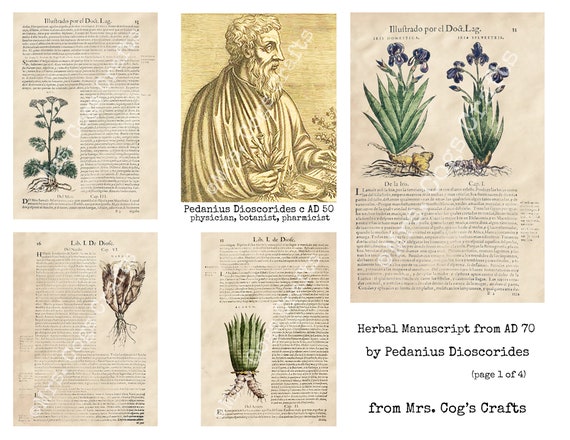The image displays a collection of five pages from an ancient herbal manuscript dating back to 70 AD, attributed to Pedanius Dioscorides, a renowned physician, botanist, and pharmacist. The pages vary in size and feature a yellowish, aged appearance with intricate etchings and black, text beneath the illustrations, though much of the writing is too small to decipher clearly. 

Page one exhibits an image of Pedanius Dioscorides himself, clad in a robe, with a long beard, meticulously examining books and flowers. His title and roles as a physician, botanist, and pharmacist are inscribed next to his figure. This page has a prominent yellow background. 

The second, third, and fourth pages showcase different botanical illustrations. Page two features a green plant with brown roots depicted underneath. Page three illustrates another green plant without flowers, while page four presents a green plant adorned with vibrant purple flowers. 

To the right of these pages, a caption notes "Herbal Manuscript from A.D. 70 by Pedanius Dioscorides, Page 1 of 4, from Mrs. Cogg's Crafts." The overall arrangement of the pages appears to be a type of product display, emphasizing their historical and botanical significance.